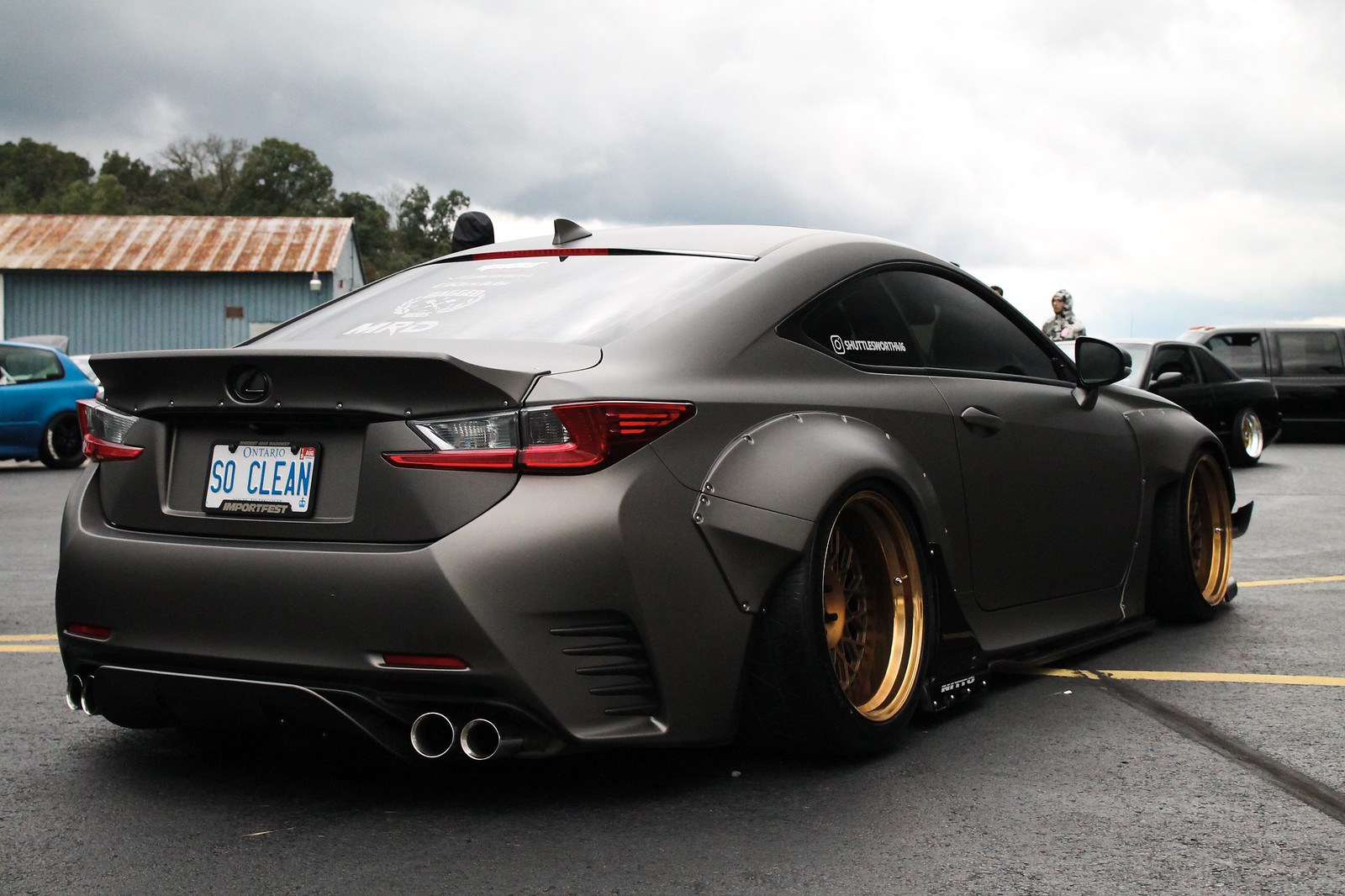In this outdoor photo, the main subject is a sleek, matte dark gray sports car, specifically a spruced-up Lexus. The car features striking gold rims and is positioned towards the back of the image. The black Lexus logo sits prominently on the spoiler, while a distinctive white license plate with light blue text reads "SO Clean" and indicates Ontario. The backdrop includes a blue building with a rusted roof on the left, and various other parked cars, including two black cars and one blue car. The sky above is overcast with dark clouds, adding to the dramatic ambiance of the scene.